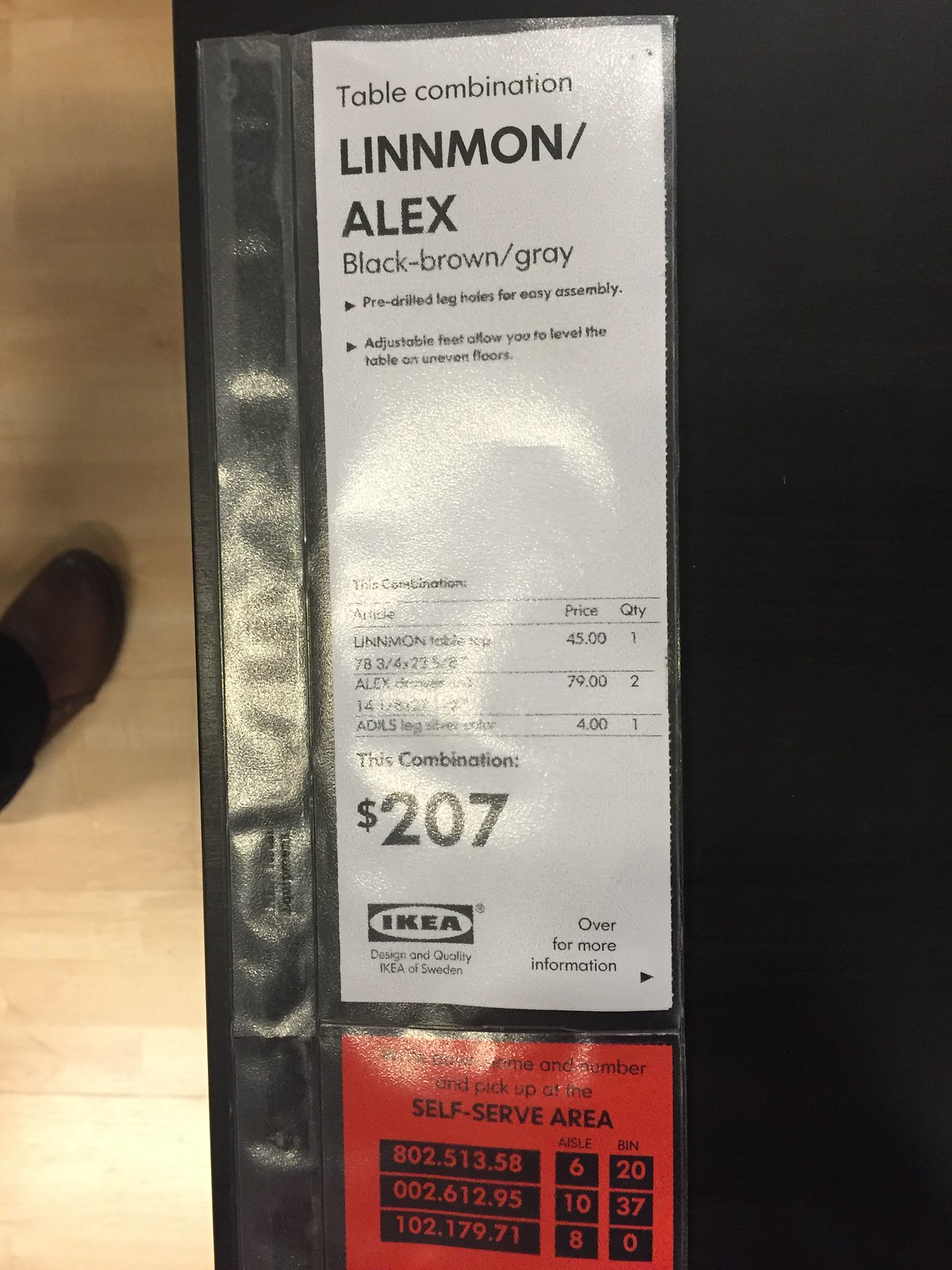The image depicts an Ikea price label on a light wood floor, partially occupied by a foot in a brown shoe on the left edge. The right side features a black background with a white, rectangular label encased in a clear protective sleeve. The top of the label reads "Table combination, LINNMON/Alex, black, brown, gray." Below, bullet points highlight key features: "pre-drilled leg holes for easy assembly" and "adjustable feet allow you to level the table on uneven floors." The price of the combination is marked as $207, but there's a reflection obscuring some of the detailed pricing information. The lower part of the label displays the Ikea logo with the text "Design and quality Ikea of Sweden." Further down, a red section with a glare indicates "self-service area" and lists specific aisle and bin numbers, though some details are hard to discern due to the glare.